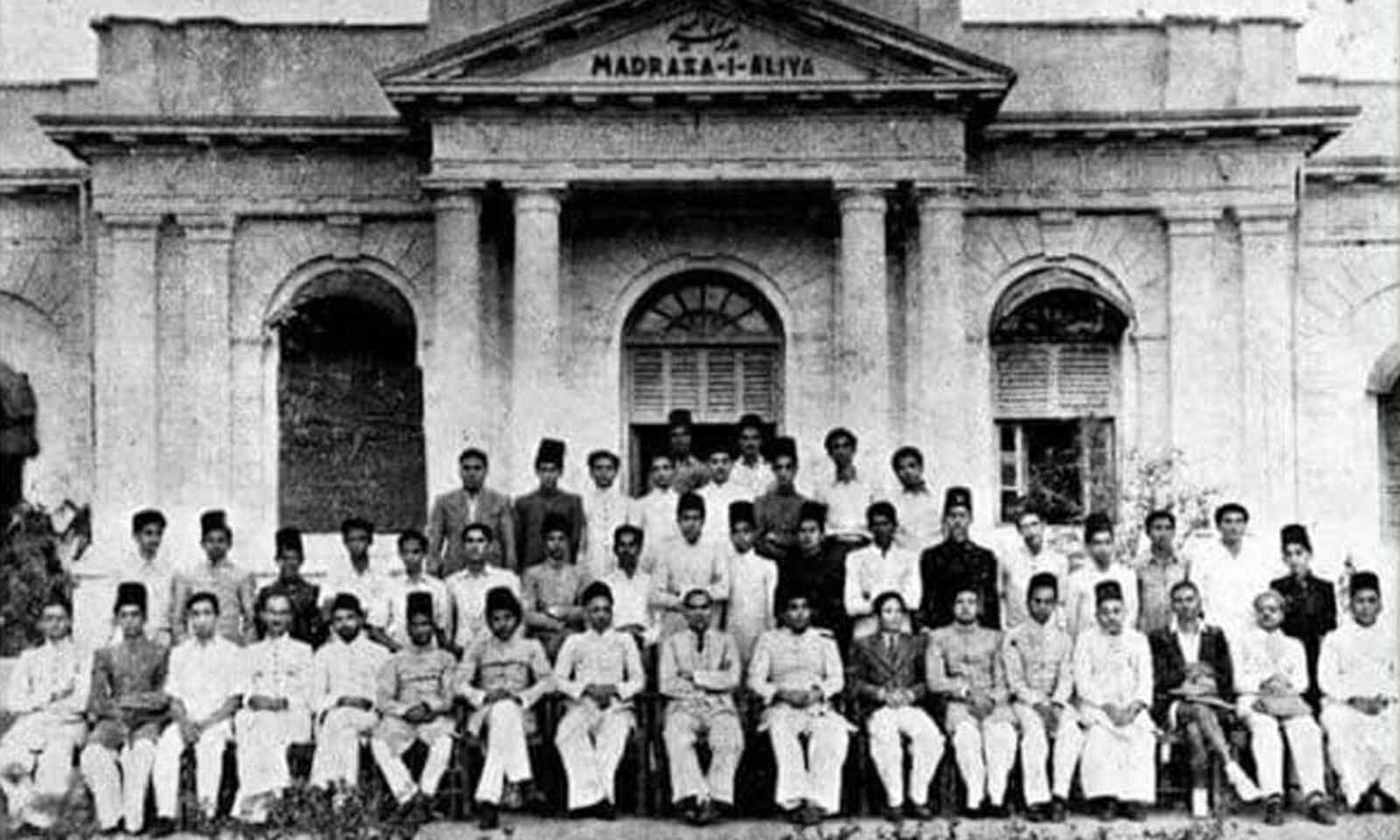The grainy black-and-white photograph captures a group of approximately 30 men posed in front of a large, stately building. The men are organized into four rows: the front row features about 15 men seated in chairs, mostly wearing white pants and seemingly official hats reminiscent of Shriners' fezes. The second row follows with another 15 men standing, dressed in a mix of white and dark suits. The third row tapers to around eight men standing, and finally, the fourth row peaks with two men standing at the top. All men stare directly into the camera with serious expressions, arranged on steps leading up to three arched doorways framed by imposing columns. Above these doorways, the text "Madraza-i-Aliya" is inscribed, though its exact origin and meaning are unclear due to the photograph’s age and poor quality.